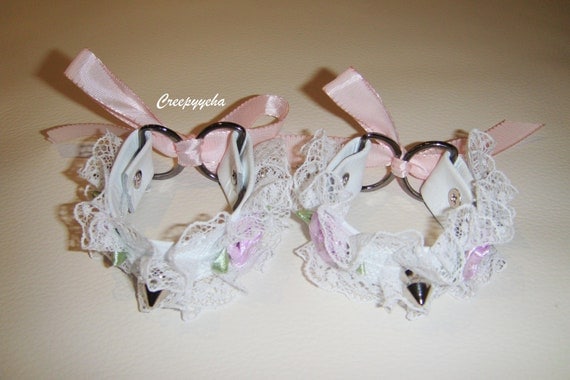The image depicts two identical decorative objects centered in a vertical rectangular frame, set against a tan backdrop that gradually lightens towards the bottom. Each object features a U-shaped structure with a flat top, adorned with white lace layered over a base, embellished with delicate pink cloth flower buds and small green leaves. At the top, two black rings or bars face each other, connected firmly by a light pink satin ribbon tied into a neat bow. The bottom of each U-shaped ornament ends in a small, black metallic cone that tapers into a sharp point. The objects may be garters or chokers and include an inscription "Creepy Echa."